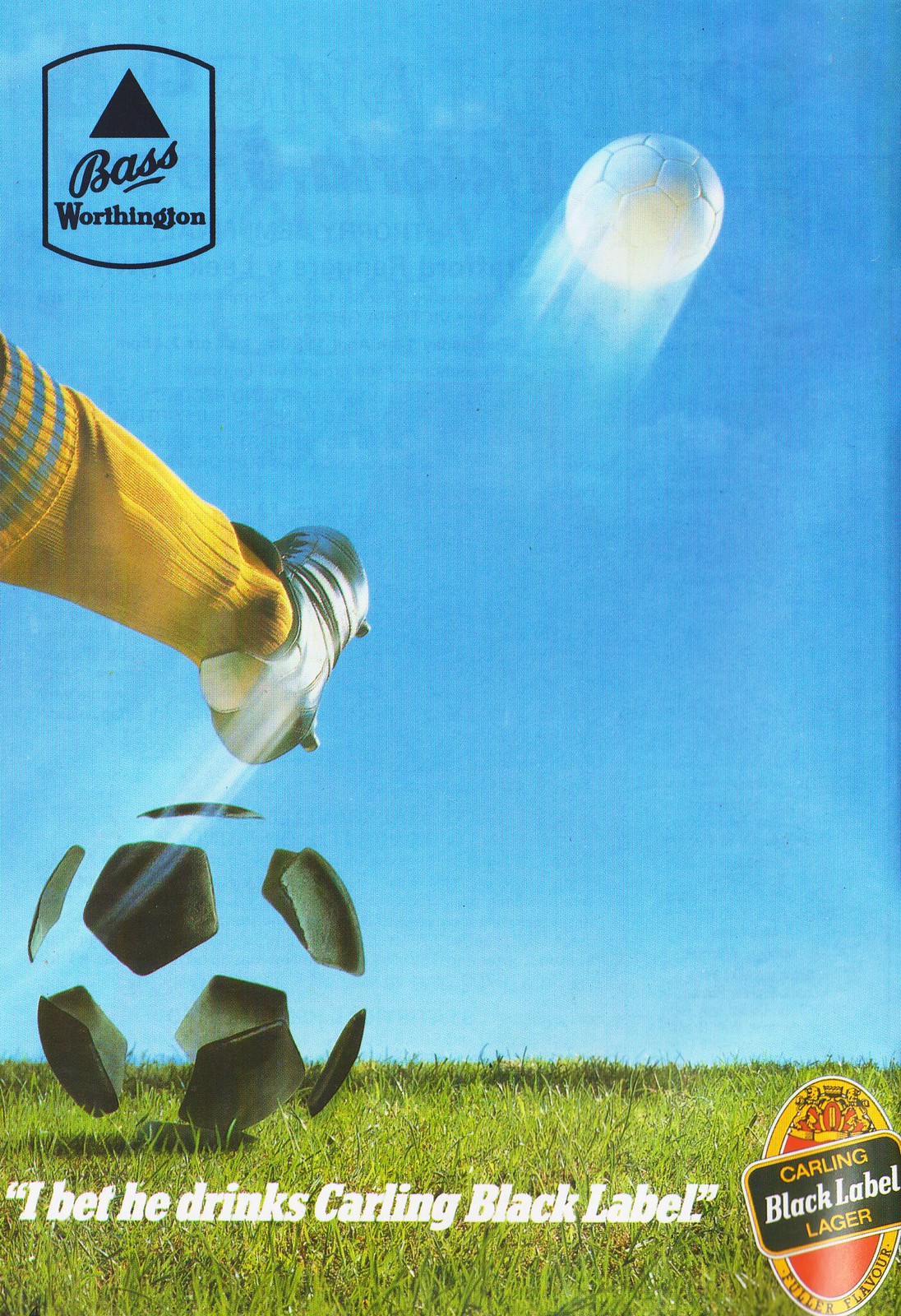This vintage advertisement from a magazine, likely from the 1970s or 1980s, promotes Carling Black Label Lager, featuring the slogan "I bet he drinks Carling Black Label" in white text on a grassy strip at the bottom. The scene captures a soccer player mid-kick, with one cleat-shod foot raised above a soccer ball. In an artistic twist, the black patches of the soccer ball are left floating in their original position on the grass, while the rest of the ball is seen soaring into the blue sky. The Bass Worthington logo is prominently displayed in the upper right corner, and the Carling Black Label logo, gold with a crown insignia, is located at the bottom right. The overall design conveys a nostalgic vibe, evoking memories of classic British beer ads.